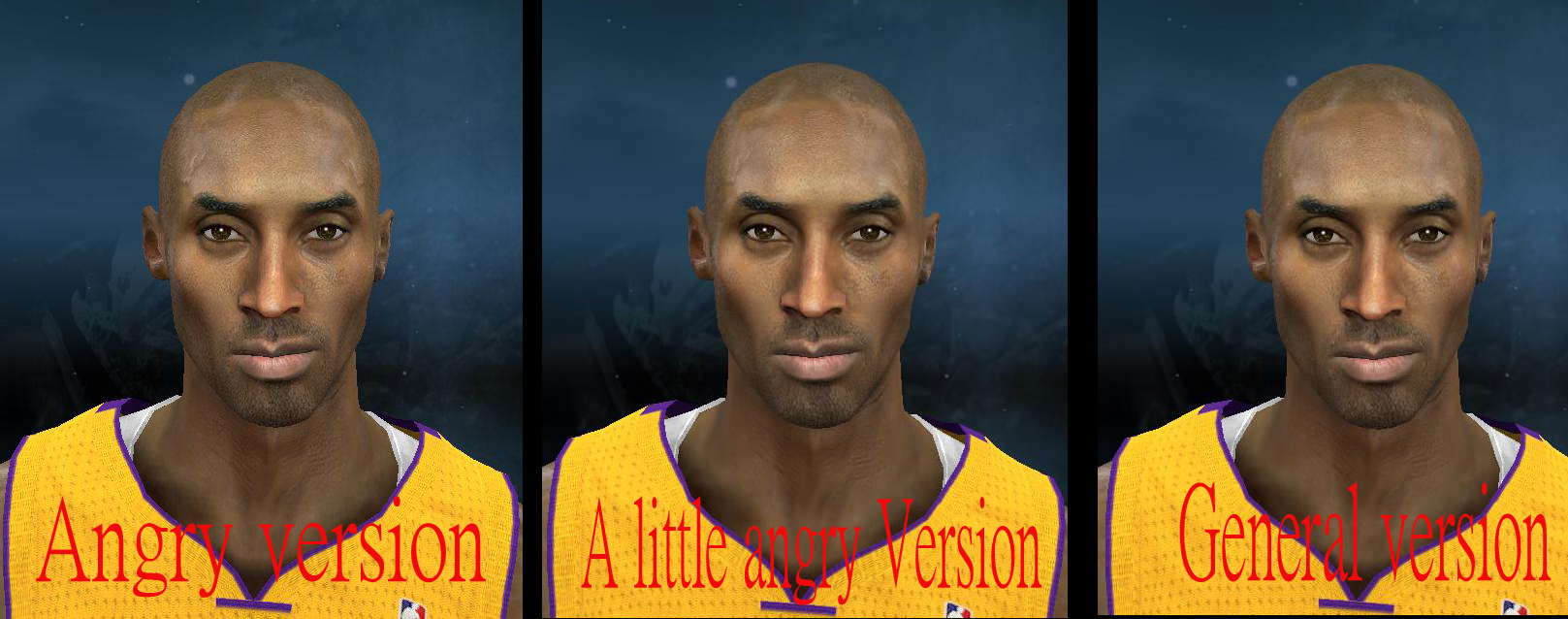This image is a meme featuring three identical computer renderings of Kobe Bryant, reminiscent of the create-a-player feature in the NBA 2K video game series. Each rendering shows Kobe in his iconic yellow Lakers jersey with purple trim, standing against a backdrop of dark blue with smeared color variations. The meme humorously labels each rendering with large, bright red text: "Angry Version" on the left, "A Little Angry Version" in the middle, and "General Version" on the right. Despite the different labels, Kobe's expression remains exactly the same in each version, reinforcing the joke that his demeanor does not change. The renderings are separated by black lines, further emphasizing the uniformity of his expressions across the different versions.